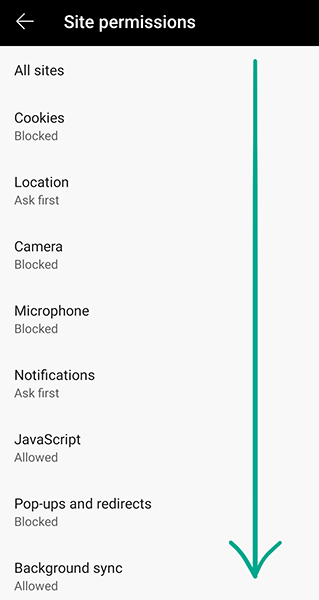This is a screenshot, likely taken from a mobile phone, as indicated by its rectangular orientation, being taller than it is wide. The top section of the screenshot features a black background spanning about an inch in height. On the far left of this black section, there is a left-pointing arrow, and centrally aligned, there's a bold text in white stating "Site Permissions." Below this title, the background shifts from black to a light gray.

Running along the right edge of the screen, about an inch from the side and extending from just beneath the black border to the bottom, is a long teal-green arrow, pointing downward.

On the left side of the screenshot, various permission settings are listed in black text:

- "All sites" appears at the top.
- Beneath it, "Cookies" is listed, followed by the status "Blocked."
- Below, "Location" is entered, with the status "Ask first."
- Under "Location," "Camera" is listed as "Blocked."
- "Microphone" follows, also marked as "Blocked."
- After a small gap comes "Notifications," with the status "Ask first."
- Underneath "Notifications," "JavaScript" is mentioned with "Allowed."
- Continuing downward, "Pop-ups and redirects" appear, marked as "Blocked."
- Finally, "Background sync" is listed at the bottom with the status "Allowed."

There is about a two-inch gap between the text and the teal-green arrow on the right. The arrowhead splits into two points, one directed upward to the right and the other upward to the left.